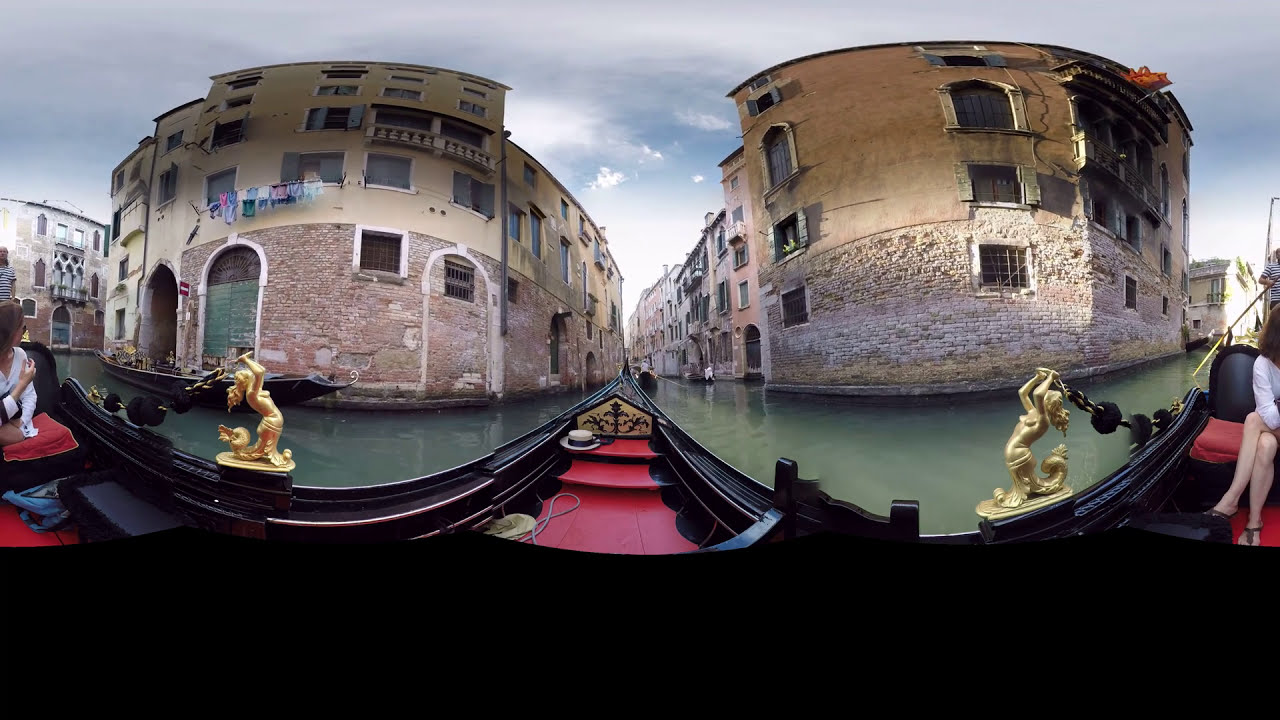The photo captures a detailed scene of a gondola navigating through the historic canals of Venice, Italy. The gondola, constructed from dark-colored wood, glides on the greenish waters surrounded by old brick buildings that partially submerge in the canal. The boat boasts an elegant red flooring accentuated with a black trim, and features a striking golden mermaid statue bending backwards on its side. Inside the gondola, a woman with brown hair, donned in a white button-up shirt and a black skirt with strappy shoes, sits cross-legged on a red cushion.

The fisheye lens effect of the image distorts the scene, giving a doubled or warped appearance. On the left side of the image, a building with a brick foundation sports a clothesline with laundry hanging outside a window. The sky overhead is mostly cloudy with hints of blue breaking through. This atmospheric shot beautifully encapsulates the charm and antiquity of Venice's age-old waterways and historic architecture.